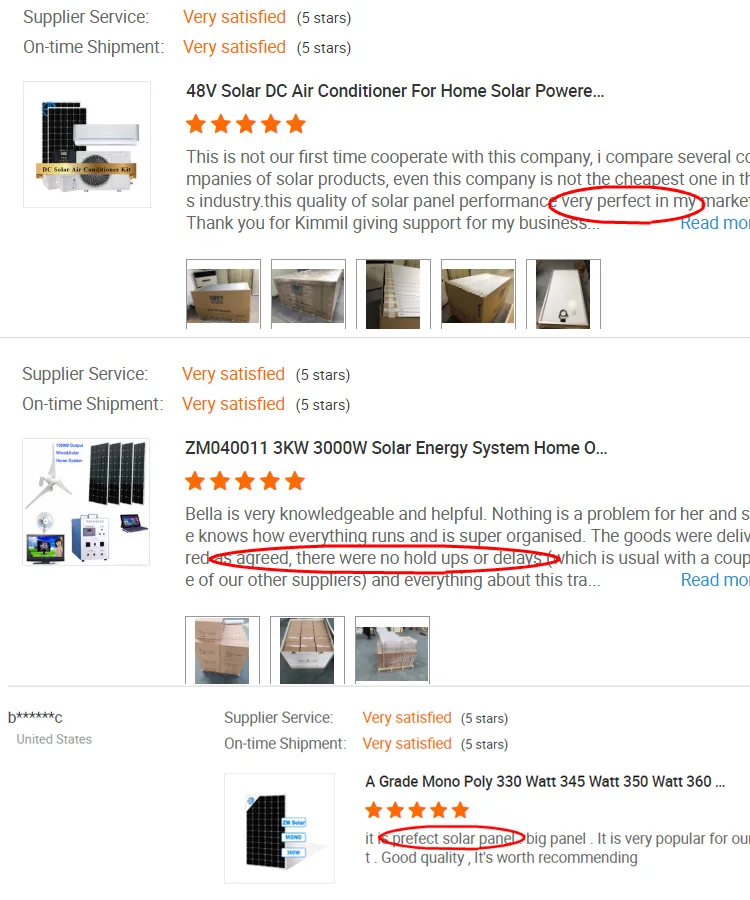The image showcases a series of reviews on a website regarding various solar power products. 

At the top, there is a review titled "Supplier Surface," accompanied by a five-star rating and the comment, "Very satisfied with five stars on-time shipment, very satisfied with five stars." The review specifically mentions a "48-volt solar DC air conditioner for home, solar powered," rated with five stars. The reviewer states, "This is not our first time cooperating with this company. I compared several companies of solar products." Despite not being the cheapest option in the industry, this company offered the highest quality solar panel performance, which proved to be "very perfect" for their market. The reviewer expresses gratitude to Kim Lee for supporting their business. Notably, the phrase "very perfect in my" is highlighted with a red circle in this part of the review. The review is accompanied by five images showing the box in which the product was shipped.

Another review continues below, again showing a five-star rating for "Very satisfied supplier service" and "Very satisfied on-time shipment," specifically for the product "ZM040011 3-kilowatt, 3,000-watt solar energy system home." The reviewer praises Bella for her knowledge, helpfulness, and organizational skills, noting, "Nothing is a problem for her, and she knows how everything runs and is super organized." Additionally, the goods were delivered as agreed, without any delays—a point emphasized with a red circle around the phrase "agreed. There were no holdups or delays." This review includes three images of the box packaging.

The final review highlights the solar panels, rated with five stars for "Very satisfied supplier service" and "Very satisfied on-time shipment" for "A-grade monocrystalline 330-watt, 345-watt, 350-watt, and 360-watt solar panels." The product is described as "perfect," and specifically noted for being a "big panel" that is highly popular and of good quality. The reviewer concludes, "It's worth recommending," with the phrase "perfect solar panel" circled in red.

The cumulative details from all reviewers highlight a high level of satisfaction with both the products and the service provided by the company.